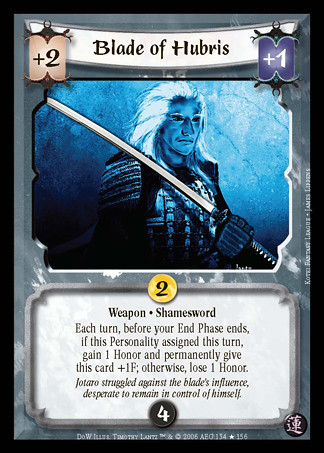This is an image of a collector's playing card from a game, intricately designed with various elements. The card features a black border and is sectioned into three distinct areas. At the top, against a white banner, the card name "Blade of Hubris" is prominently displayed in black text. Flanking this title, on the left side is a tan decal with "+2" and on the right side, a purple decal with "+1".

Dominating the middle section is a striking, blue-tinted illustration of a samurai-like man with long, flowing white hair. He holds an impressive sword and wears detailed armor, including shoulder pieces and gloves, looking fiercely to the right.

Below this central image, the card provides gameplay instructions and narrative details on a white background with black text. Key gameplay information includes a gold circle with the number "2" and a black circle with a white "4". The text describes the weapon "Shamesward," with instructions on honor mechanics in the game, followed by a flavor text: "Jotaro struggled against the blade's influence, desperate to remain in control of himself."

In the card's bottom section, small print includes the name "Timothy Luntz 2005," various numbers, a star, and a sequence "156." There is also a circle on the bottom right featuring characters written in either Japanese or Chinese, adding to the card's exotic theme.